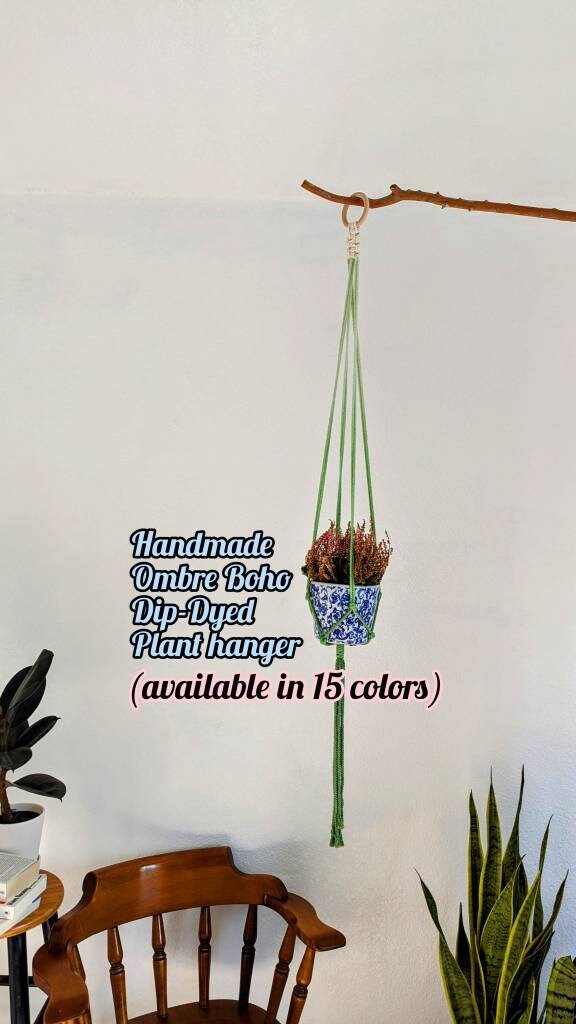The image showcases a beautifully arranged interior scene with an emphasis on a handmade ombre boho dip-dyed hanging planter. The planter itself is a striking combination of a white background adorned with a blue floral pattern. It is suspended from an orange branch by four green ropes that wrap around the base, ending in ornamental tassels. The small plant within the planter features eye-catching reddish-orange leaves. 

Beneath this central hanging feature, a white wall serves as a backdrop with blue text outlined in black stating, "Handmade Ombre Boho Dip-Dyed Plant Hanger," followed by black text with a pink outline that reads, "Available in 15 Colors." Adding to the room's decor are a wooden chair with slatted back, a wooden stool topped with a book and another planter, and additional plants with tall, thick, dark green leaves positioned behind them. The overall setup creates a harmonious and inviting atmosphere, making it clear that this is an advertisement for a stylish and unique hanging planter available in a variety of colors.